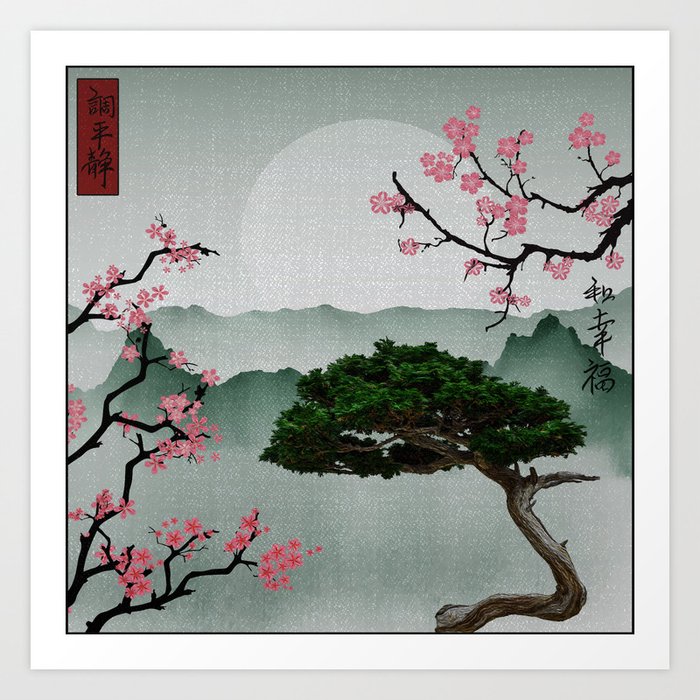The framed painting, mounted on an off-white wall, is an intricate piece with distinct Asian influences, possibly Japanese or Chinese. The painting features a large, pale moon or sun against a gray sky, with rows of gray mountains below. Dominating the foreground is a large bonsai-like tree with a gnarled, S-shaped, gray trunk that twists toward the top, where a lush canopy of green leaves spreads out. At the bottom right of the painting, the tree's trunk and branches extend in various directions. Adding to the serene scene are pink flowers blooming on brown branches, positioned in both the top right and bottom left corners of the painting. Notably, a vertical red rectangle with Asian characters in dark ink is present in the top left corner, and similar characters appear halfway down on the right side, partially obscured by the tree's branches. The painting’s border includes a white frame with a narrower black-lined border inside of it. The textured canvas gives the artwork an almost fabric-like appearance, enhancing its depth and detail.